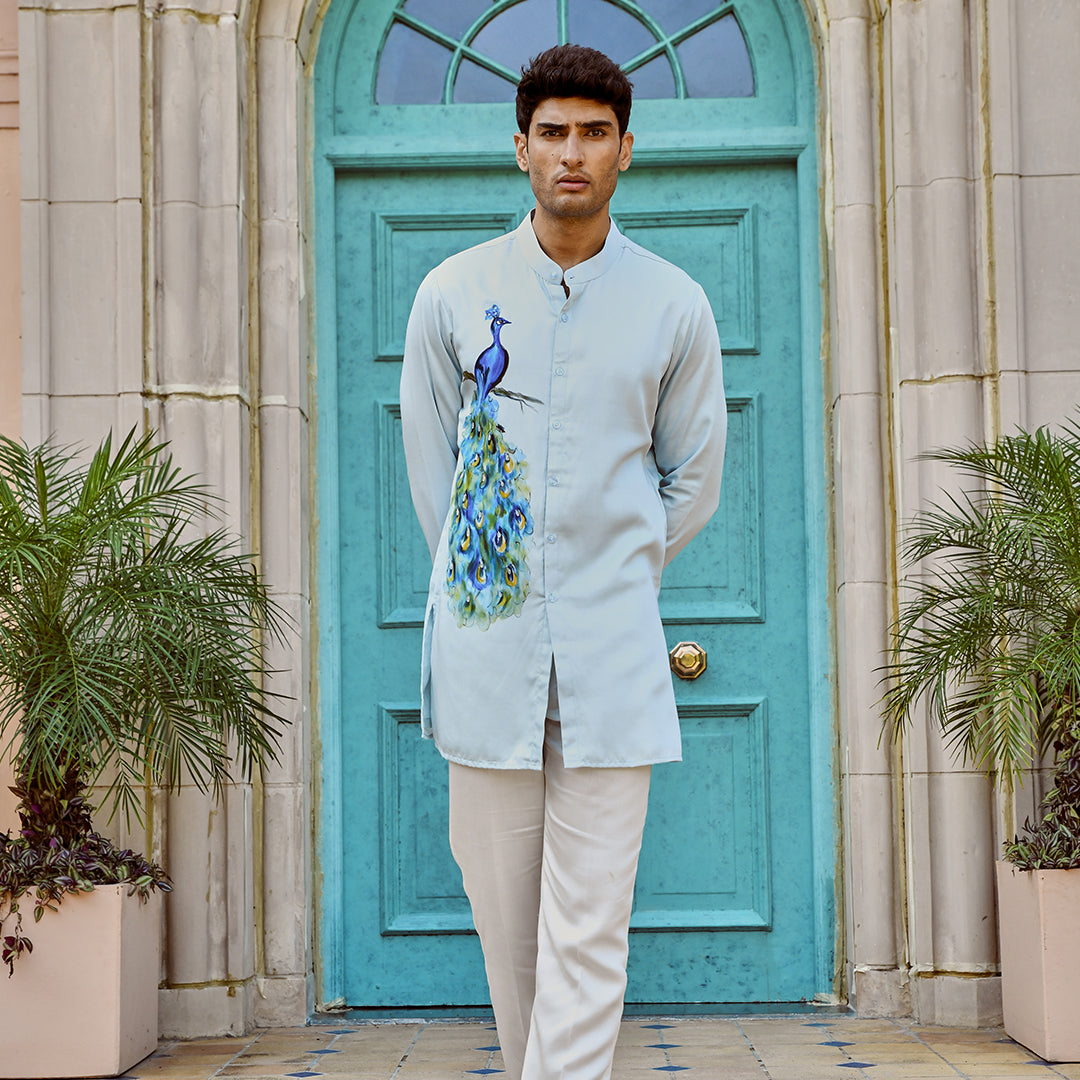In this color photograph, a young man, appearing to be in his late 20s to early 30s and possessing Indian or Middle Eastern features, stands outdoors during the day. He is centered in a square-format image, modeling a light blue tunic shirt that falls just below his waist. The shirt, which is long-sleeved with a stand-up collar and buttoned up the front, features an intricate embroidery of a peacock on the left chest. The peacock, perched on a branch, displays its long, colorful tail feathers, rich with the characteristic "eyes," cascading down the shirt. The man, with dark, short hair, stands with his hands behind his back, exuding a sense of calm poise.

He is situated in front of an antique-looking blue door with a Palladian arched window. The door, accompanied by a visible gold doorknob near his hip, is framed by cream-colored stucco walls and concrete pillars. The man stands on an off-white and blue diamond patterned floor, with potted green plants flanking either side of the doorway, adding a touch of nature to the scene. The overall setting suggests a mix of architectural elegance and fashion, potentially aimed at a stylish or social media-savvy audience. The photograph embraces a realistic and representational style, capturing both the subject and the surroundings with vivid detail.